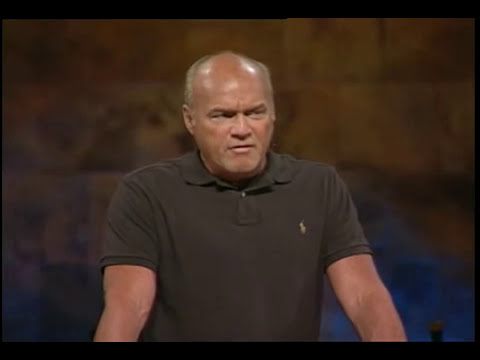In the center of the image stands an older, middle-aged man, approximately in his 50s, with pronounced male pattern baldness and some gray or blonde hair on the sides. He is wearing a brown short-sleeved polo shirt with a visible Ralph Lauren logo on the top right corner. The man is depicted from just below the elbows and up, with his arms tensed and extended outward, suggesting he is leaning on them. His expression appears serious, concerned, and slightly surprised. He is oriented towards the viewer but gazes off to the right side of the image (the five o'clock direction). Behind him is a blurred brownstone wall made of large, rectangular stone blocks, potentially indicating an indoor setting that could resemble a stage or a public place. There are faint blue lights visible at the bottom of the wall, adding to the impression of a stage-like environment, where the man seems to be reacting to something out of frame. The overall color palette of the image includes shades of brown, tan, black, and white.